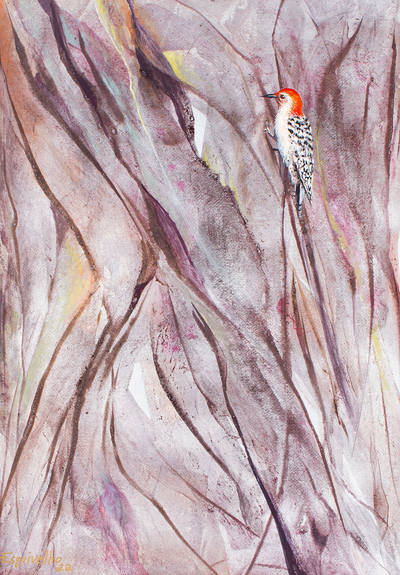This image features a detailed painting of a bird set against an abstract, impressionistic background that resembles a textured tree trunk. The background is dominated by various brown and blackish patterns that run vertically from the bottom to the top, mimicking branches. These patterns are interspersed with softer swipes of colors like blue, mauve, orange, and yellow, adding depth and a subtle complexity to the scene. The background also features some raised, ridged textures, enhancing the impression of a natural but abstract environment.

Positioned about an inch down from the top and an inch from the right, the bird sits gracefully on one of these brown branches. It is facing left, with its back turned to the right. The bird's head is a striking orange, contrasted with white around its eyes extending down its stomach. It sports a black beak and black eyes, while its back is adorned with a mix of black and white spots. The tail feathers also display this black and white pattern, and the bird's wings exhibit a grayish-white tone with similar black spots. Overall, the scene artfully combines vibrant and subdued tones to create a dynamic yet harmonious portrayal.